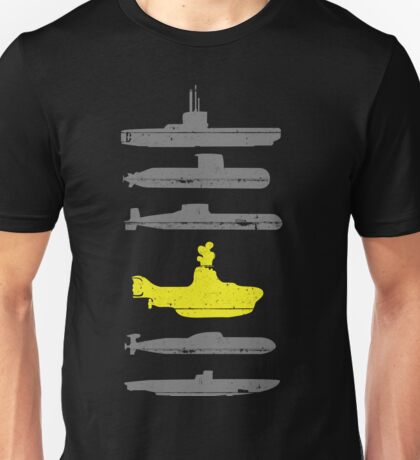This color photograph showcases a close-up view of a Caucasian man's upper torso, adorned in a dark gray, short-sleeved t-shirt with a crew neck. The t-shirt is the focal point of the image, filling the frame almost entirely, and is set against a clean, white background. The man's pale arms are positioned at the bottom left and right corners of the image, with his neck and collarbone visible at the top, though his head is not shown.

Central to the t-shirt's design are a series of naval vessels, specifically submarines, rendered in gray and yellow. Starting from the top and progressing downward, there are three gray submarines followed by a distinct, bright yellow submarine that bears a resemblance to the iconic Beatles' Yellow Submarine, complete with what appears to be smoke or steam emanating from its top. Below the yellow submarine, two additional gray submarines are depicted. This orderly vertical arrangement creates a striking contrast between the subdued gray tones and the vibrant yellow, lending visual interest to the garment. The image gives the impression of a professional stock photo, likely intended for use on a t-shirt retail website, with no text present on the shirt itself.